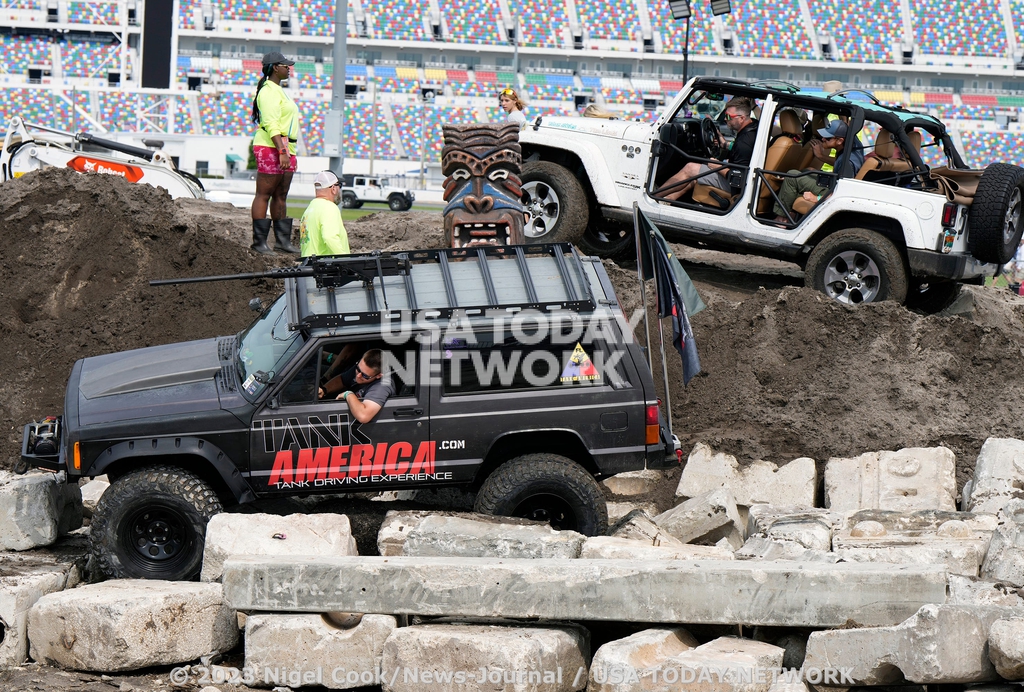In this color photograph, we see a dynamic off-road scene featuring two utility vehicles in action on a dirt track. In the foreground, a dark gray vehicle with large wheels is navigating a rugged path lined with large stones. The driver, a man with dark hair and glasses, is wearing a short-sleeved gray shirt and has his left arm casually hanging out of the window. The vehicle is branded with "TankAmerica.com Tank Driving Experience" and features a rifle mounted on its roof and flags attached to its back. 

In the middle ground, standing on a dirt mound, are two individuals in fluorescent green shirts overseeing the vehicular activities. Accompanying them is a tiki-style carved totem with distinct Polynesian features, adding an eccentric touch to the setting.

In the background to the top right, another vehicle, white in color, is visible. This four-door off-road jeep, moving in a different direction, has no doors and is filled with a family of four, all clad in a mix of shorts, pants, and dark tops. Behind this white jeep is a distant audience appearing as colorful dots in yellow, red, and white, reminiscent of spectators in racetrack bleachers.

At the very bottom of the image, a text label reads "2003 NIGEL.COOK / NEWSJOURNAL / USA TODAY NETWORK" in white. The scene vividly captures both the adventurous spirit of off-road driving and the vibrant atmosphere of the event.